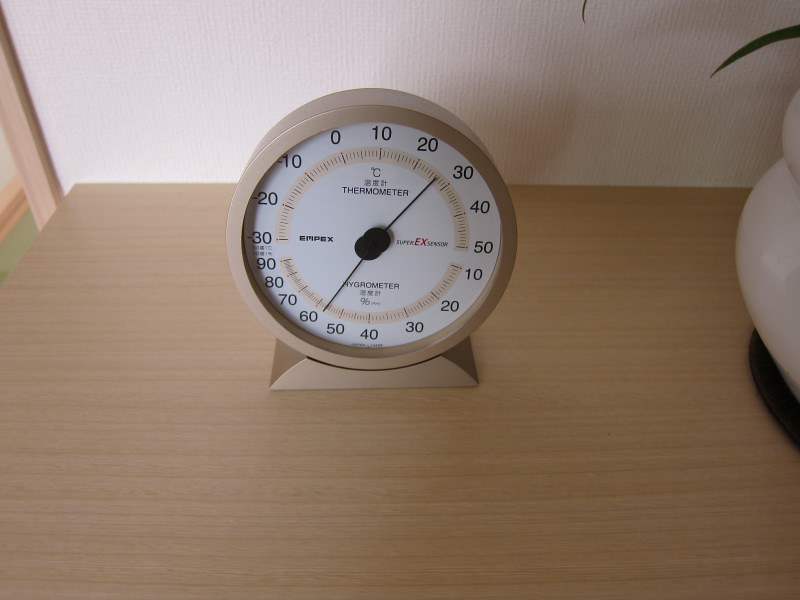This horizontal photograph showcases a somewhat vintage-looking thermometer with a circular face, exuding a nostalgic charm. The body of the thermometer is a soft beige color, complementing its placement on a pale wooden tabletop, which appears to be an end table or perhaps a bedside table. The thermometer's face is white, enclosed by an inner beige ring that features detailed temperature markings. The dark matte black hands, with thin needles, precisely point to the current temperature and humidity levels. 

In the thermometer, the hygrometer is positioned at the bottom while the thermometer occupies the top portion. Both instruments measure in Celsius, with the hygrometer indicating relative humidity as a percentage. The brand, MPEX, is known for its Super EX Sensor, prominently noted on the right side of the device. Presently, the thermometer reads 26 degrees Celsius and indicates that the room's humidity is slightly above 55%.

The lighting in the setting is muted, casting a subtle shadow onto a lighter beige, textured wall in the background, which enhances the vintage ambiance of the scene.